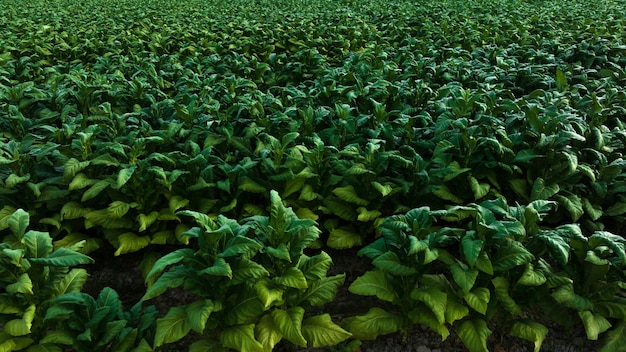The color photograph depicts a densely packed field of green, leafy plants, likely tobacco or a similar crop, growing outdoors on a farm. The plants, which cover the entire image, feature large, wide, and triangular leaves that cluster together, creating a lush and uniform appearance. Each plant stands approximately a foot tall, although the exact height is difficult to gauge. There's visible soil scattered throughout, emphasizing the farmland setting. The close-up perspective reveals no buds, fruits, or flowers on the plants, suggesting they are in an early growth stage. The arrangement appears bushy and full, potentially organized in rows, although this is not clearly visible.